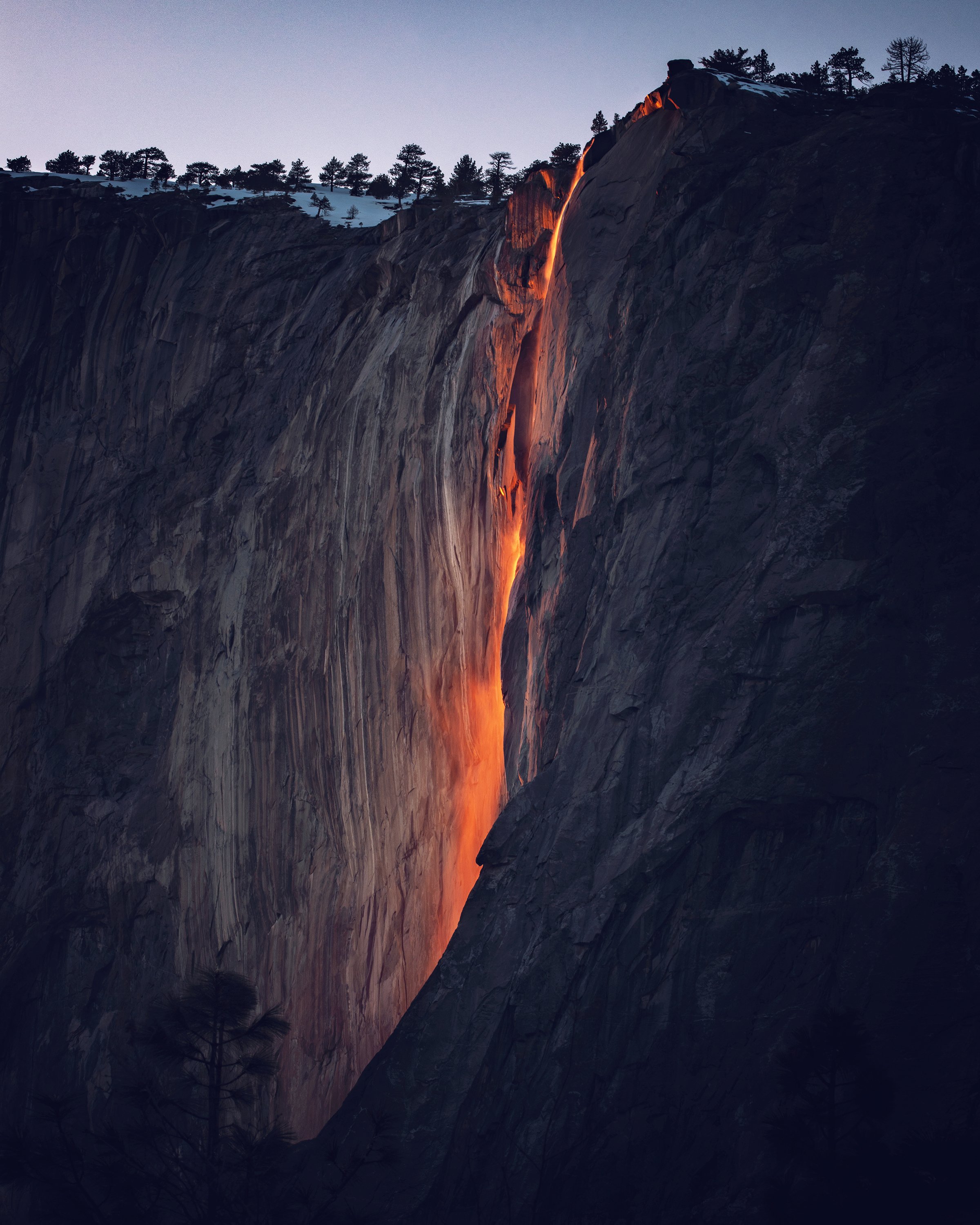This striking photo, possibly digitally enhanced or naturally captivating, captures the phenomenon known as Fire Falls in Yosemite at dusk. The image features a towering, dark cliff adorned with snow and fir trees at its summit, juxtaposed against a twilight sky transitioning to night. A narrow stream, resembling flowing lava due to the sun’s orange afterglow, cascades down a cleft in the mountainside. The bright, medium-orange hue of the falling water creates a fiery appearance that illuminates the surrounding rock face, adding a mystical glow to the scene. Despite the dark and shadowy backdrop of the cliff, the misty, luminous fall stands out vividly, rendering a mesmerizing blend of natural beauty and optical illusion.